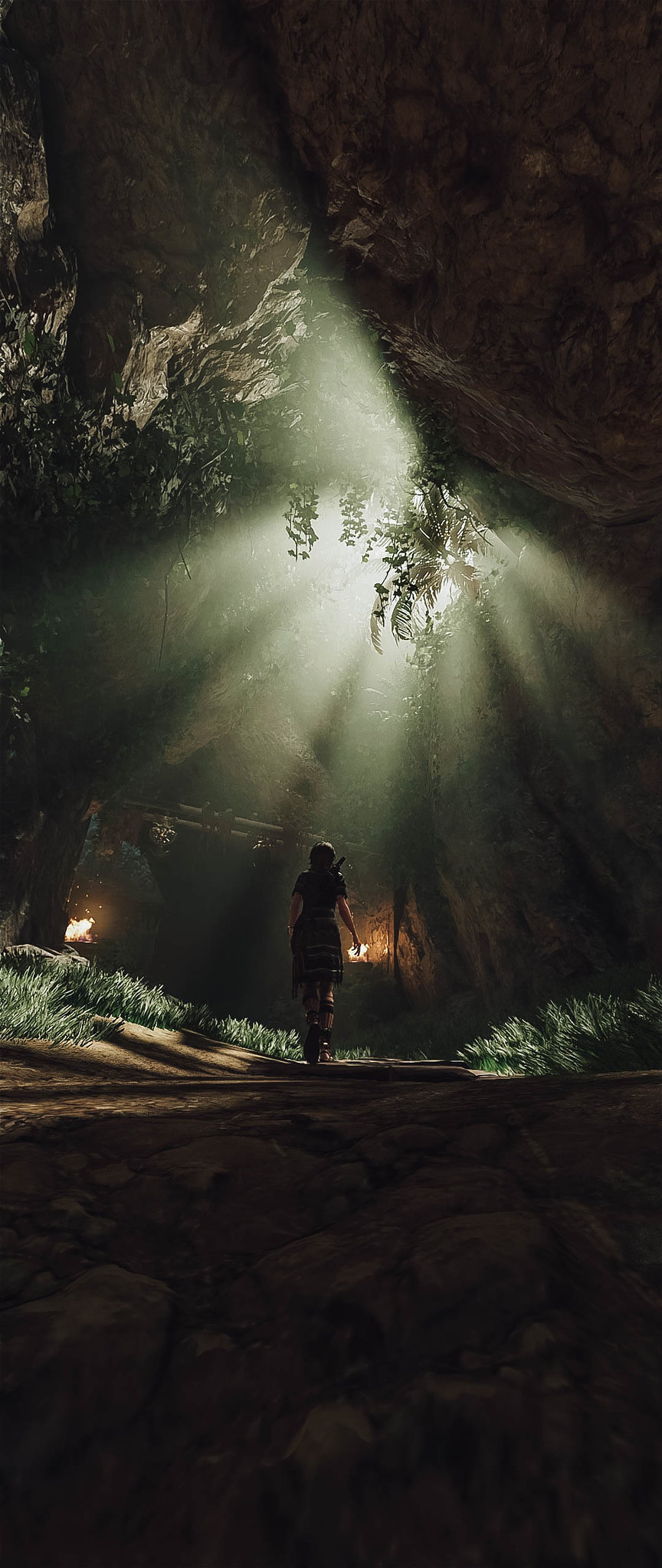The image resembles a scene from a computer game and is tall and narrow in format. The foreground, occupying the bottom third of the frame, is dominated by dark brown and black hues, which on closer inspection, reveal the rugged outlines of rocks. At the horizon line, a female character is seen walking away from the viewer on a dirt road, flanked by short, sage-colored shrubs or grass. To her left, there is an entrance resembling a cave or temple, framed by flames on either side to illuminate the path. Above the entrance, the sun's glare shines brightly through a dense tree line, casting a pronounced white light with tree tendrils visible around it. In the upper left corner of the image, a rocky cliff face begins to emerge, suggesting that the character is exploring a mountainous region.